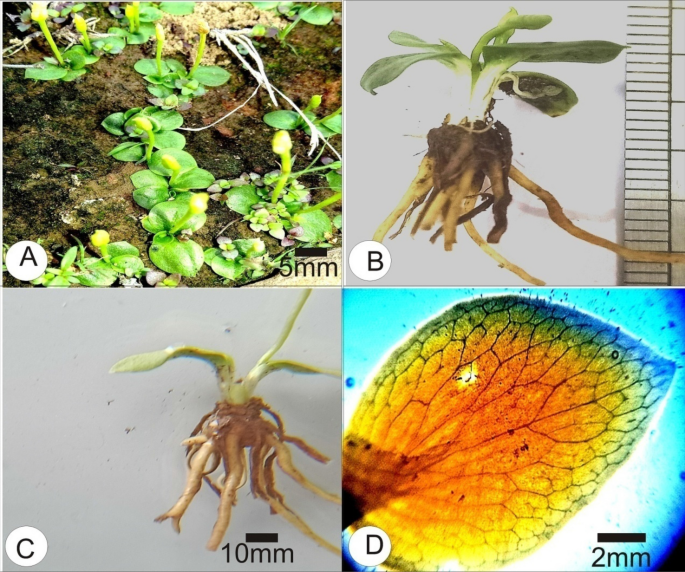This image contains a grid of four scientific diagrams labeled A, B, C, and D, each providing detailed views of plant structures and scales for measurement. 

In the top left corner, Diagram A features an area of soil with small green plants growing, some of which have yellow flowers. A scale at the bottom indicates a measurement of 5 millimeters. Diagram B, in the top right, presents the roots of a small plant set against a white background with green leaves sprouting from the top; a ruler is positioned along the right side for reference.

The bottom left, Diagram C, shows another plant with its roots fully exposed and three green leaves; this diagram includes a scale reading 10 millimeters at the bottom. Finally, Diagram D on the bottom right displays a magnified view of a leaf, highlighting the intricate vein structure in various colors: blue on the edges, transitioning to green, and then orange in the center. This close-up is accompanied by a scale marked at 2 millimeters. Overall, the image appears to be part of a detailed scientific study showcasing different aspects and measurements of plant anatomy.